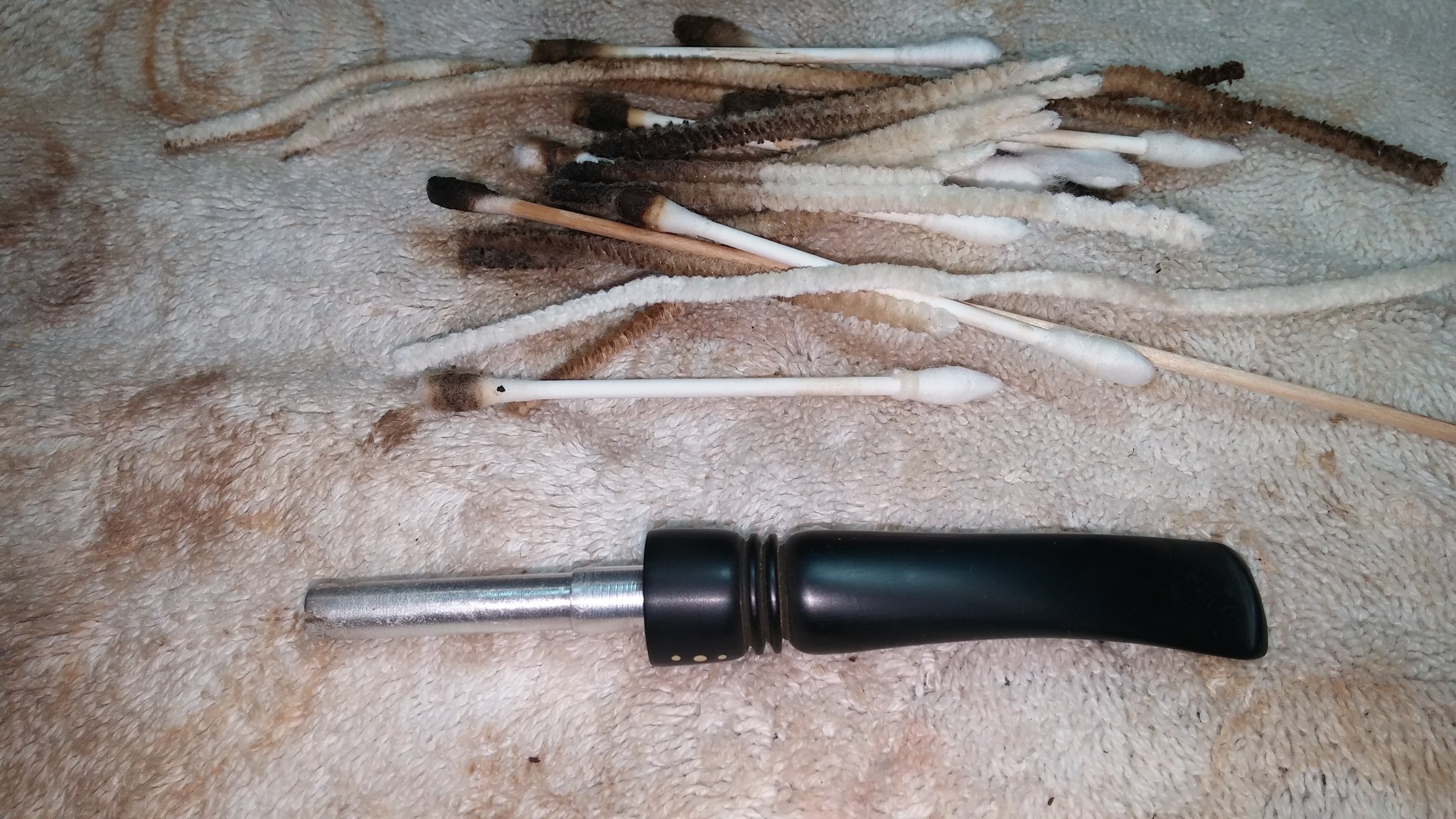The image captures a detailed scene on a modeled, marble-like countertop featuring white and brown hues. Prominently positioned at the bottom center is a black-handled tool that resembles a screwdriver designed to accommodate various bits, although no bit is currently inserted. This tool, which may be plastic or wooden, has a silver tube extending from the handle. Above the tool lies a messy heap of approximately 15 dirty Q-tips and pipe cleaners. The Q-tips and pipe cleaners, which are slightly bent and stained with brown and black soot or debris, are mostly clean on the right side but get progressively dirtier towards the left. Notably, one Q-tip in the center is distinguished by its exceptionally long wooden handle. The scene suggests an indoor setting, possibly with the camera’s flash activated, adding brightness to the environment. The surface beneath these objects, mistaken at first as a garment or blanket due to its furry texture, is actually part of the countertop and shares the countertop's stained appearance.